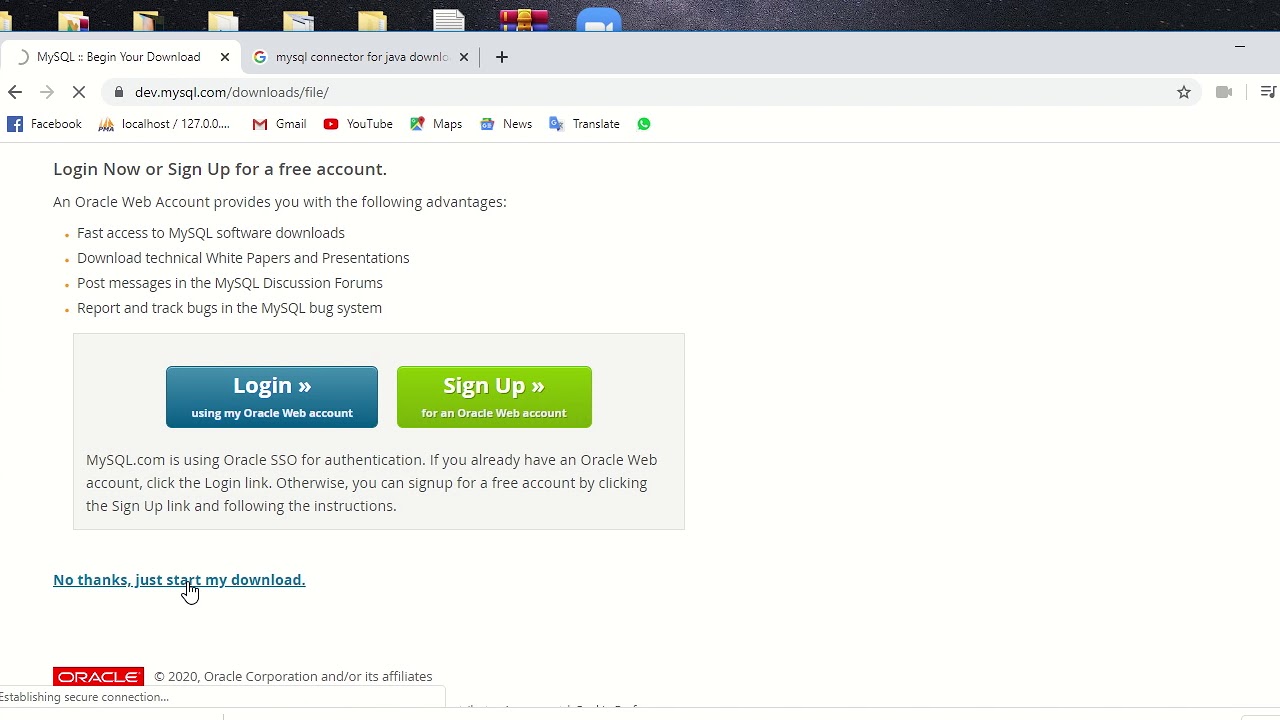The image depicts a Windows computer screen displaying a Chrome browser with two open tabs. The active tab is on the "MySQL - Begin Your Download" page, hosted by Oracle. The web page appears somewhat dated with a plain, white background. Prominently in the center, there are large "Log In" and "Sign Up" buttons. Underneath, the page highlights the benefits of creating an Oracle web account, such as fast access to MySQL software downloads, the ability to download technical white papers and presentations, post messages in discussion forums, and report and track bugs. However, at the bottom of the page, there is a discreet link labeled "No thanks, just start my download," which allows users to download MySQL without creating an account.

The second tab, visible in the browser, is related to the first and shows a page titled "MySQL Connector for Java Download." Along the bookmarks bar in the browser, several saved bookmarks are visible. These include shortcuts to popular sites like Facebook, Gmail, YouTube, and Google Maps, as well as a bookmark titled "Localhost," presumably used for local web development.